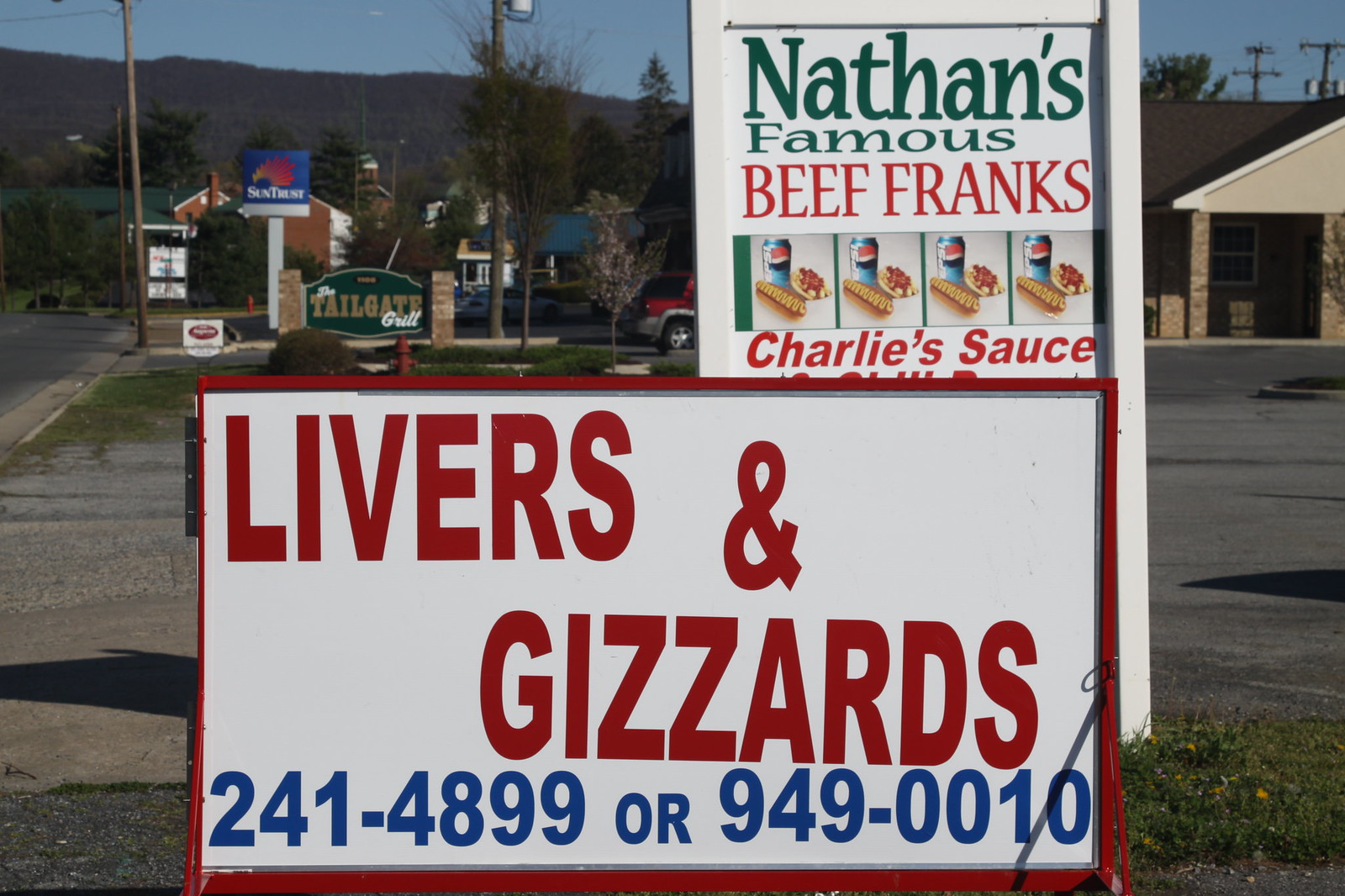In this outdoor scene set in what seems to be a small town or suburban area, two prominent signs catch your eye. The first, closest to the camera, is a large white sign with bold red lettering advertising "Livers and Gizzards" along with phone numbers in blue. Directly behind this, there's a second large sign promoting "Nathan's Famous Beef Franks" featuring a series of images depicting hot dogs paired with cans of Pepsi and mentioning "Charlie's sauce." The surroundings include a paved parking lot near small buildings, possibly a restaurant or hotel with signs reading "Tailgate" and "Seafood" in blue and red. In the backdrop, the scene is enriched with a scattering of little trees, parked cars, a road, and distant mountains, all framed by a grassy area, evoking the charm of a quiet, less commercialized locality.